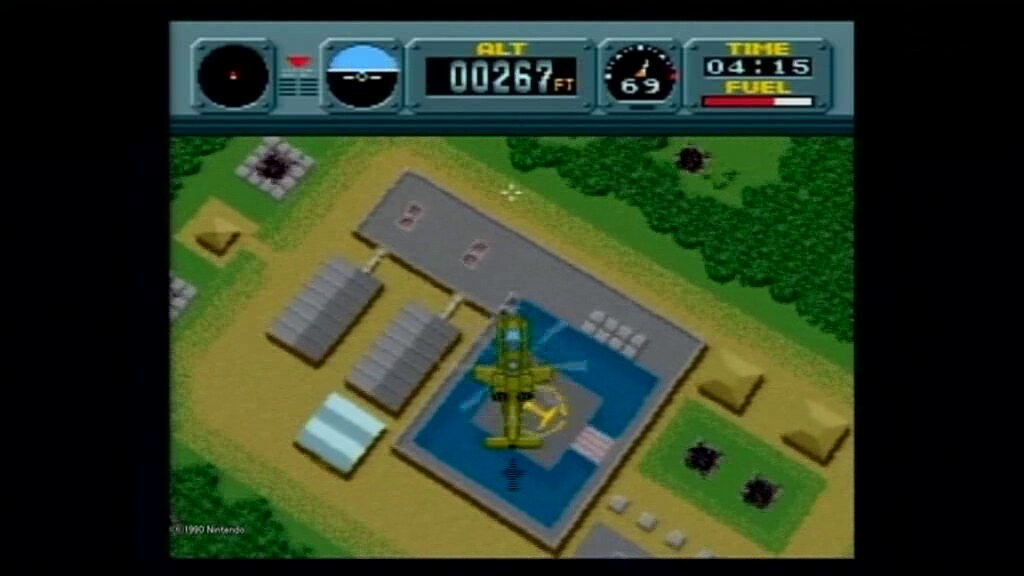The game screenshot showcases a helicopter, resembling an Apache model, hovering over a complex on an older-style overworld map. This game, created by Nintendo and copyrighted in 1990, features a retro visual style with flat structures and minimal depth. The complex below consists of a central helipad, which is square and blue, surrounded by buildings, including gray sheds, and green spaces filled with trees. The helicopter, primarily green and designed for one or two occupants, is shown floating above this helipad. At the top of the image, there's a detailed user interface displaying various metrics: a radar, a gyroscope, and digital readouts including an altitude of 267 feet, a speed of 69, and a fuel gauge mostly red indicating fuel level at 04:15. The UI also includes time, altitude, and fuel information, stylized with gray and yellow elements. The terrain below is depicted with some dirt and scattered greenery around the complex.